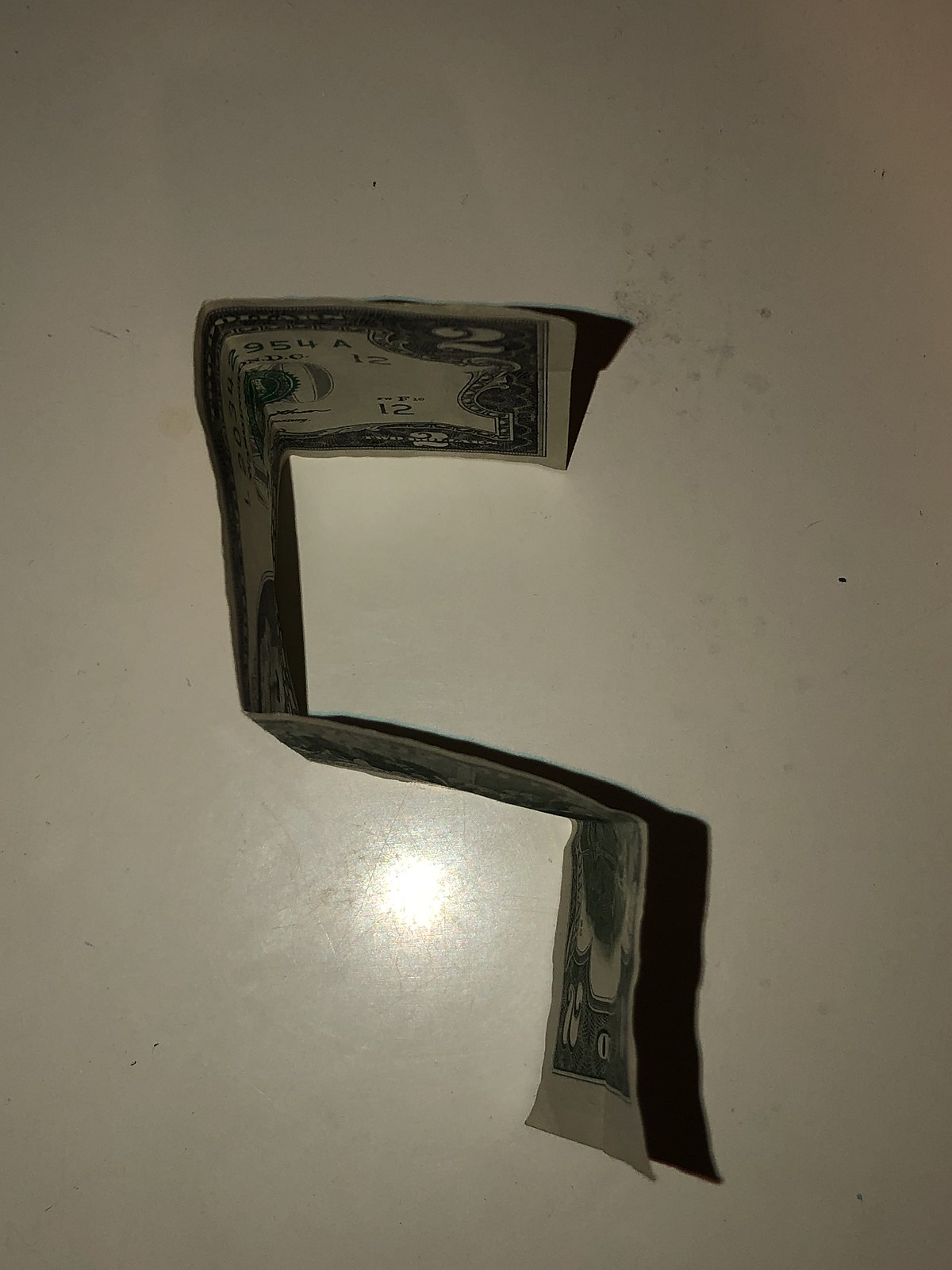The image is a color photograph depicting an intricately folded American $2 bill. The bill is folded in a distinctive S-shape and is positioned to view from the top down. Clearly visible is the "2" marking in the top right-hand corner of the bill. The folds create a series of right angles: the top section is horizontal, it then folds vertically down the middle of the image, continues in a slightly diagonal downward path towards the bottom right, and concludes with another vertical fold on the bottom right side. The folded bill casts a shadow onto the dirty white linoleum surface below. The background features a bright spot in the lower third beneath the bill, likely from the camera flash used to capture the photograph, adding a light contrast to the scene.